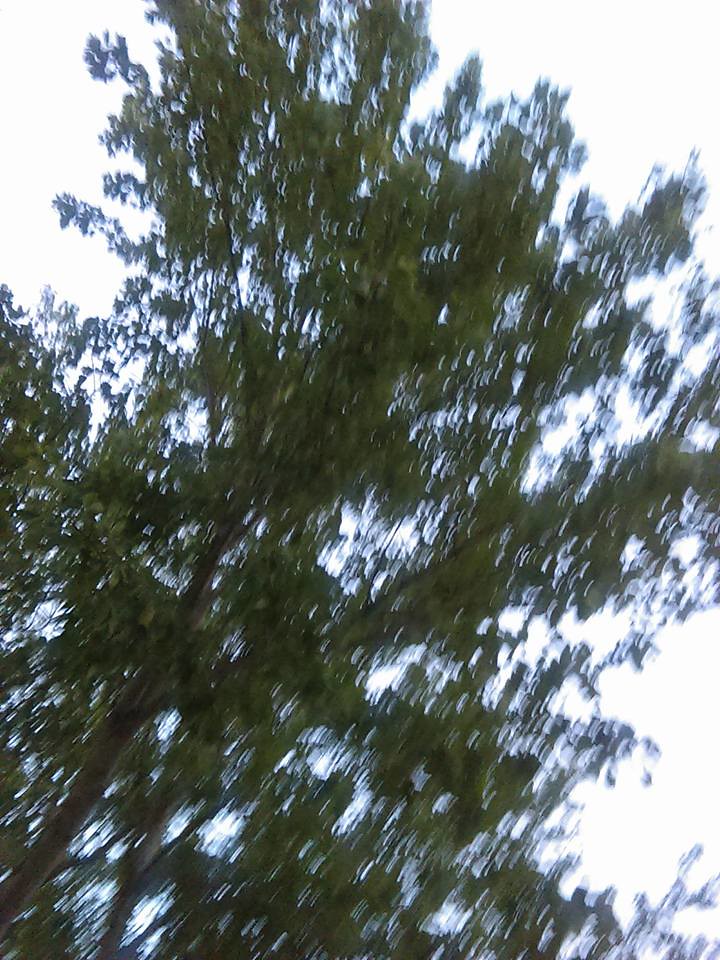In this image, we're looking upwards at a tall tree from a low vantage point. The photo is somewhat blurry, and prominently features a brown tree branch on the left-hand side with another branch visible behind it. The majority of the image, roughly 85%, is dominated by dark green leaves that densely cover the tree. Scattered throughout the foliage, there are several openings through which bright white light from the sky shines through. These openings are primarily located in the top left corner, top right corner, and the bottom right corner of the photograph. The interplay of the dark green leaves and the bright white light creates a striking contrast, emphasizing the natural beauty of the tree and the serene sky in the background.